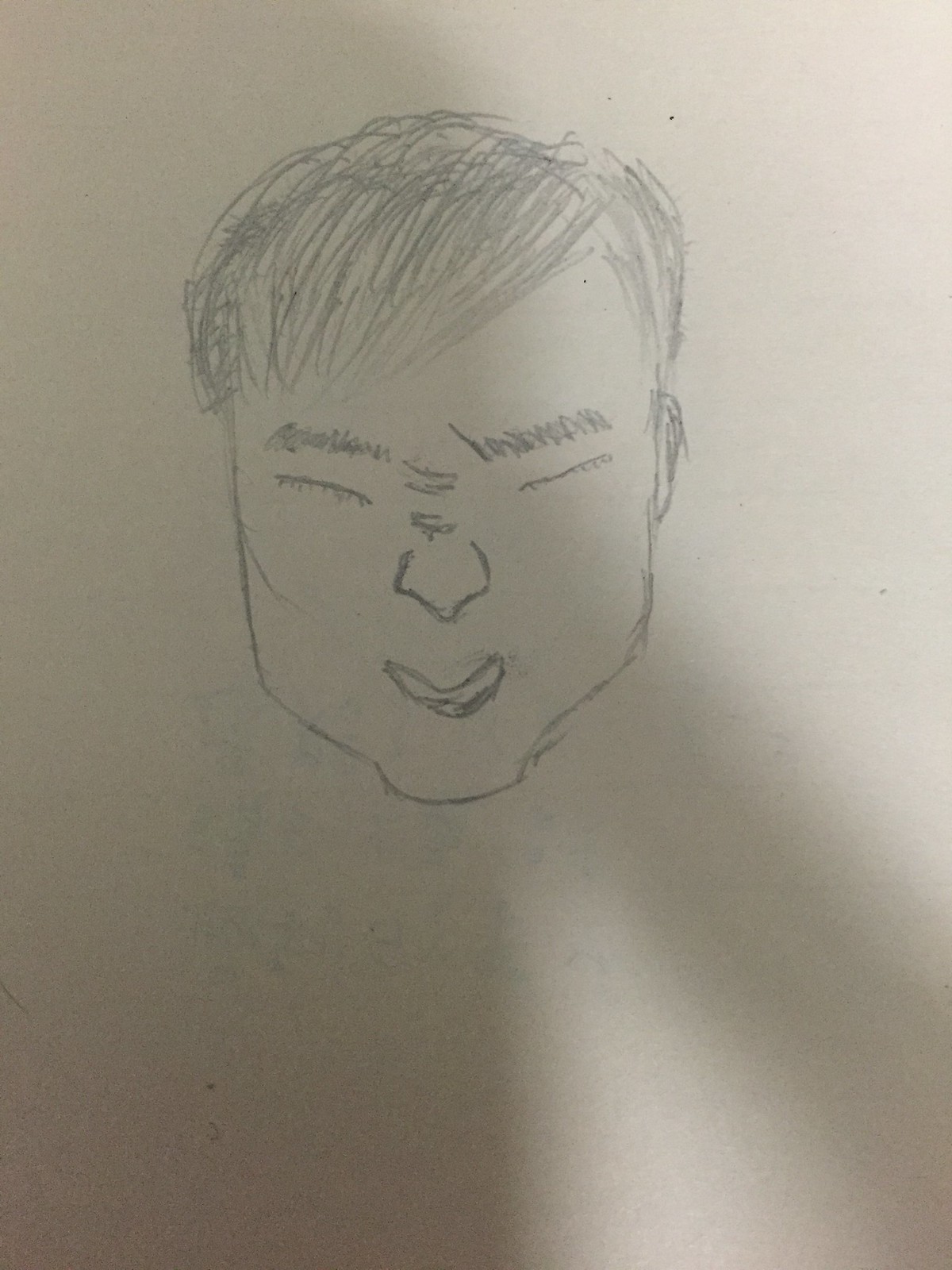The image displays a detailed pencil sketch of a man's head on white paper, with a distinct shadow falling on the left side. The man has dark hair, parted on the right with a slightly messy fringe across his forehead. His eyebrows are irregularly shaded, with the left one being narrower at the inner end and wider further out, while the right eyebrow has unusual lines sticking up, maintaining the same width. His eyes are completely closed, represented by slightly upward-slanting lines. The nose is depicted with a minimal, somewhat diamond-shaped and scribbled shading. His mouth is a curvy, smile-like shape reminiscent of a 'bubble letter U' or a 'curvy banana,' leaving the space within the lips unshaded. He has a pronounced, square-shaped jaw with a protruding chin. The drawing is simplistic yet expressive, capturing the essence of the facial features despite some crude elements.